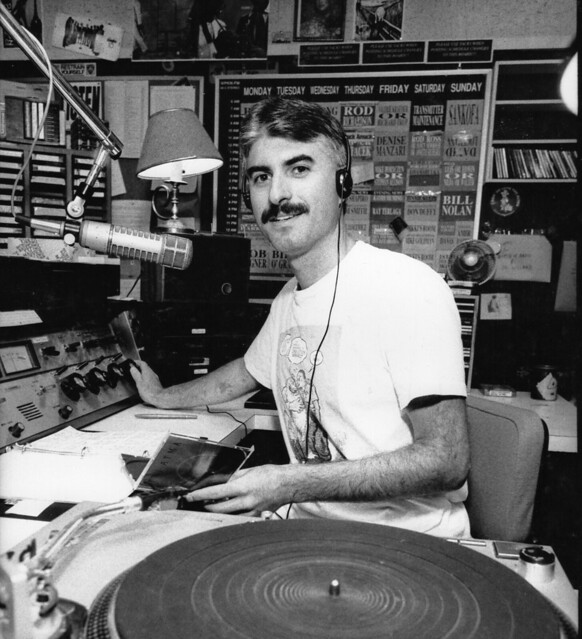The photograph is a vertically rectangular black and white image depicting a radio DJ at work in an indoor studio setting under artificial lighting. The DJ, a slightly graying Caucasian man with short dark hair and a mustache, is wearing a short-sleeve white shirt and thin, wired headphones. He is seated at a booth, and the scene is framed by the equipment surrounding him. A record player occupies much of the lower portion of the image with its black rubber mat clearly visible. The DJ is turning one of the black dials on the control panel to his left while holding an open CD case. A microphone extends from the upper left corner, and a desk lamp is positioned just behind him. The background features a playlist schedule detailing the days of the week, and rows of tapes for different commercials are scattered about. A very thin black border can be seen along the right-hand side of the photograph. The DJ looks directly into the camera, not speaking, creating a posed and contemplative atmosphere.